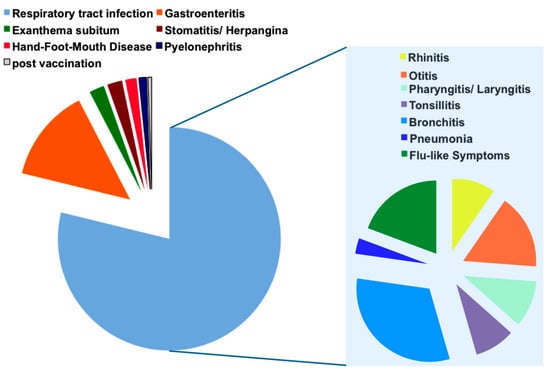This image features two pie charts, each with distinct medical data and color-coded sections. The left pie chart, set against a white background, predominantly highlights Respiratory Tract Infection, encompassing over 75% of the chart in blue. The remaining segments are assorted medical conditions: gastroenteritis, exanthema subitum, stomatitis/herpangina, hand, foot, and mouth disease, pyelonephritis, and post-vaccination effects, represented in colors such as orange, green, brown, pink, and white.

The right pie chart, on a light blue background, further disaggregates the main blue segment from the left chart into smaller sections. These include flu-like symptoms, bronchitis, pneumonia, tonsillitis, pharyngitis/laryngitis, otitis, and rhinitis. Unlike the left chart, the segments in the right chart are spaced apart, visually emphasizing each condition's part in the overall spectrum. Both charts are accompanied by legends correlating colors to specific medical conditions: 

- Respiratory Tract Infection (blue)
- Gastroenteritis (green)
- Exanthema Subitum (orange)
- Stomatitis/Herpangina (pink)
- Hand, Foot, and Mouth Disease (brown)
- Pyelonephritis (white)
- Post-vaccination effects (various smaller colors)
- Additional conditions on the right chart include rhinitis, otitis, pharyngitis/laryngitis, tonsillitis, bronchitis, pneumonia, and flu-like symptoms.

The diagrams offer an intricate view of these conditions, potentially related to broader health contexts like COVID-19 given the mention of post-vaccination.